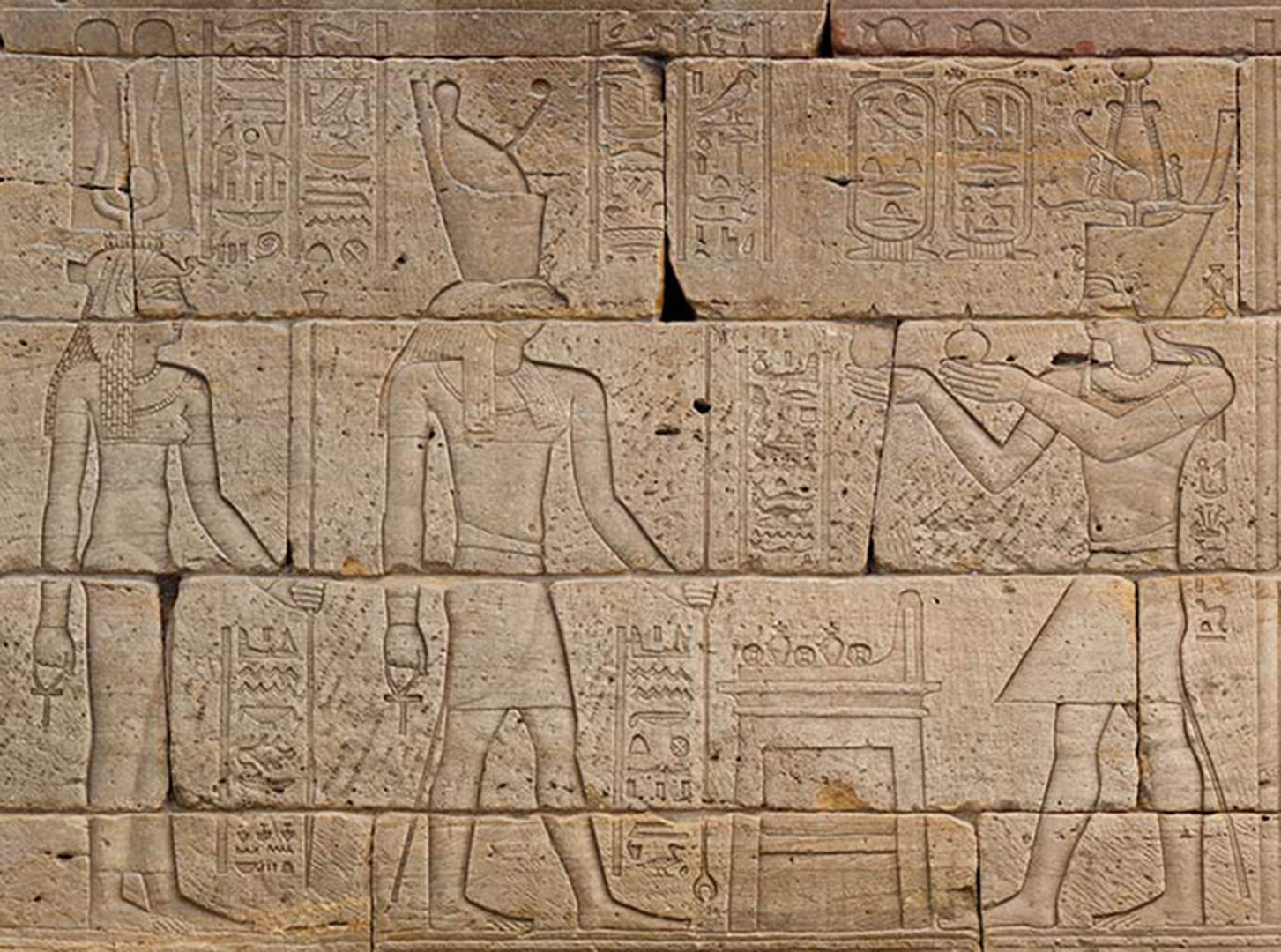The image depicts an intricate stone brick wall adorned with ancient Egyptian carvings. The background, composed of thick, tan-colored bricks suggestive of a pyramid, features hieroglyphics and detailed designs. On the left side of the wall stands a figure, likely a woman, adorned in a beaded headdress and ankle-length skirt, holding an ankh—a cross with an oval-shaped top—in her left hand. To her immediate right is a male figure donning a large headpiece and a chest piece, with a cloth wrapped around his waist that resembles a kilt or shorter skirt. He also holds an ankh. The far-right figure, similarly attired with an Egyptian-style headpiece and skirt, is depicted juggling circular objects. Beneath these figures, a surface is visible with additional circular objects resting on top. Above their heads, the brick wall features a series of intricate carvings and designs, including rectangles, squiggly lines, triangles, birds, and eyes, evoking a rich tapestry of Egyptian symbolism.